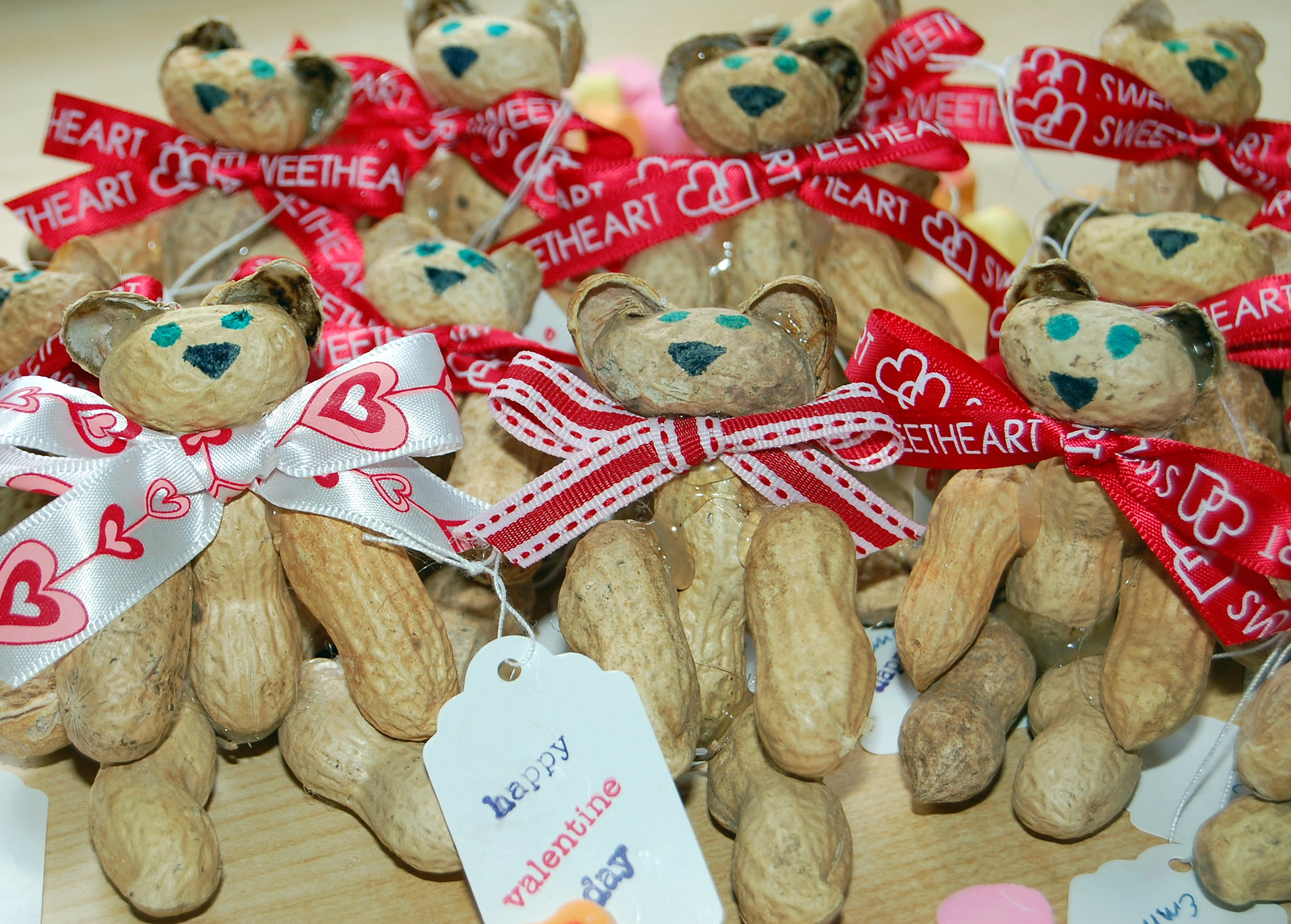In this detailed and whimsical image, numerous bears are meticulously crafted from various peanut parts. Each bear has a long peanut body, with additional peanuts ingeniously attached to form arms, legs, and heads. The heads feature green eyes and blue noses intricately drawn, adding a playful character to each bear. A mix of ribbons adorns their necks: the bear in the center sports a striking red ribbon with white edges, while the bear on the left side boasts a white ribbon decorated with red and pink hearts. The remaining bears wear red ribbons inscribed with "Sweetheart." In front of this heartwarming assembly, a tag reading "Happy Valentine's Day" is prominently displayed. All these charming bears stand proudly on a brown platform, with a softly blurred background that accentuates their intricately detailed forms.